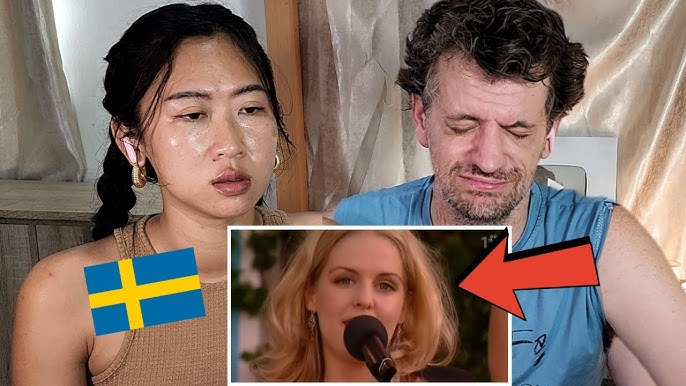The photograph prominently features two main subjects, a woman and a man, who appear to be in their 30s and 40s, respectively. The woman, positioned on the left, has an Asian appearance with long dark hair tied in two ponytails, and she wears large gold earrings and a tan sleeveless top. Her makeup is minimal but includes lipstick. She is visibly sweaty and looks exhausted. In front of her is the flag of a Scandinavian country, specifically a blue flag with a yellow cross, often associated with Sweden.

To the right stands a middle-aged Mediterranean-looking man. His hair is medium-length, black with some gray around the sides, and wavy. He's clad in a blue sleeveless shirt with the sleeves rolled up to his shoulders. He sports an unkempt beard and stubble, and like the woman, he looks tired and sweaty. Both individuals are in front of a backdrop that consists of light-colored curtains and some wooden elements.

Superimposed on the lower part of the photograph, in front of the woman, is a smaller picture frame. This inset shows a young white woman with long blonde hair talking into a microphone. She appears to be performing or speaking. A large red arrow points directly at this smaller image, drawing attention to the blonde woman.